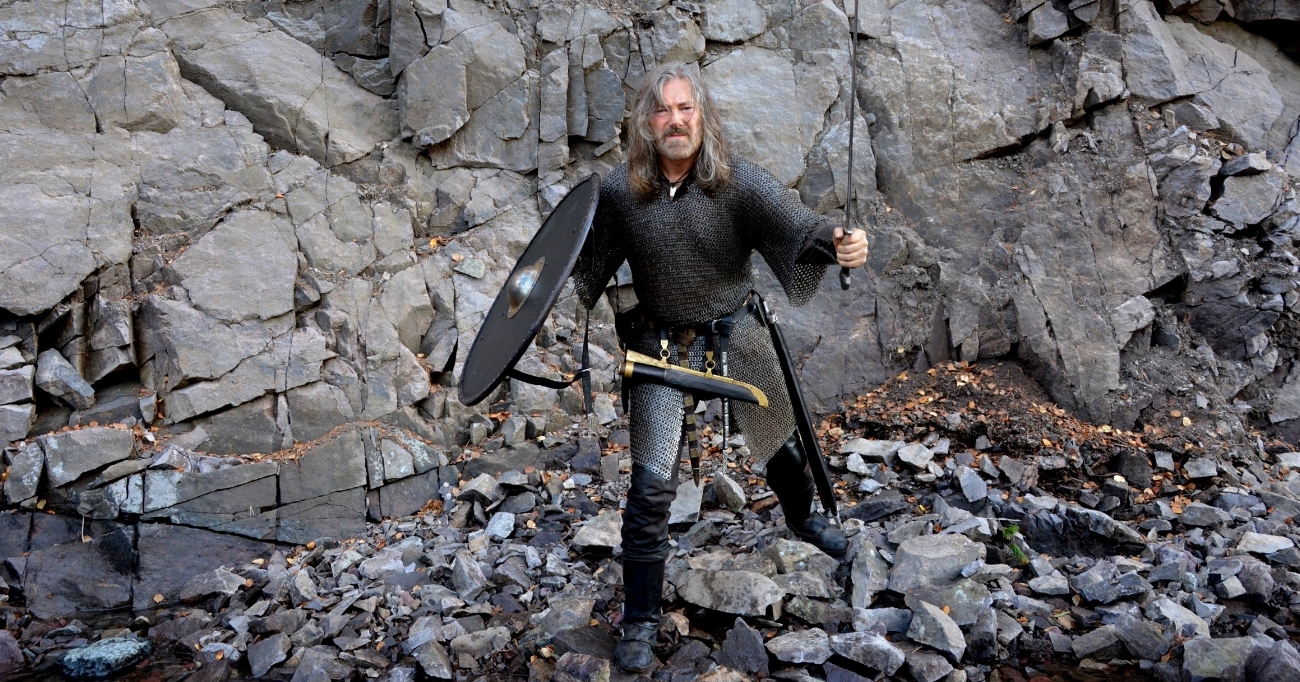The color photograph is a horizontally-oriented, detailed depiction of a man in medieval-style armor, standing against a large, gray stone cliff. The rugged rock wall forms the background, with loose rubble of the same gray stone scattered in the foreground. The man, with long gray hair and a matching beard and mustache, looks up at the viewer, adopting an aggressive stance. Clad in a dark gray chain mail shirt and leggings, he also sports black boots that rise above the knees. In his right hand, he holds up a dark bronze round shield with a pronounced silver-colored raised center, gripped by a large strap on the back. His left hand extends forward, brandishing a sword that points upward. Secured around his waist, he carries a black sword sheath, complemented by an additional dagger sheath strapped over his thigh. The photo, embodying photographic representationalism realism, captures the dramatic essence of a medieval knight poised for battle in a somber, overcast setting.